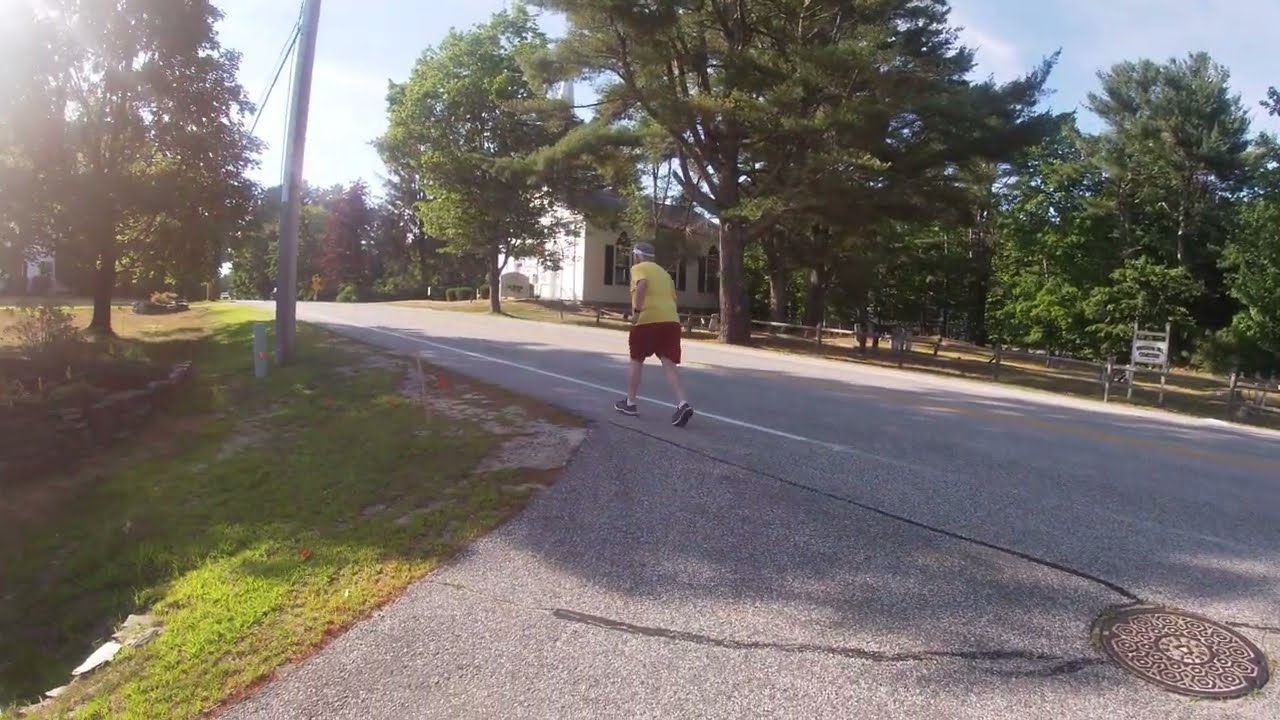In this outdoor photo taken on a sunny day with a blue sky and sparse white clouds, a middle-aged man is captured jogging along the shoulder of a road. He has gray hair and is wearing a yellow t-shirt, red shorts, white ankle socks, gray sneakers, and a white headband. The man is in motion, with his back facing the camera, running beside a white stripe marking on the pavement. The surrounding scene is vibrant with lush green grass on either side and numerous green trees in full bloom, indicative of a warm summer day. In the background, there is a white house with dark shutters and to the left, a power pole with electrical wires stretching across the sky. Additionally, a closed manhole cover is visible on the road near the bottom right of the image. There is a white sign with black writing to the far right center, though its text is indiscernible. The road itself is devoid of vehicles, enhancing the serene and pleasant atmosphere of the landscape.